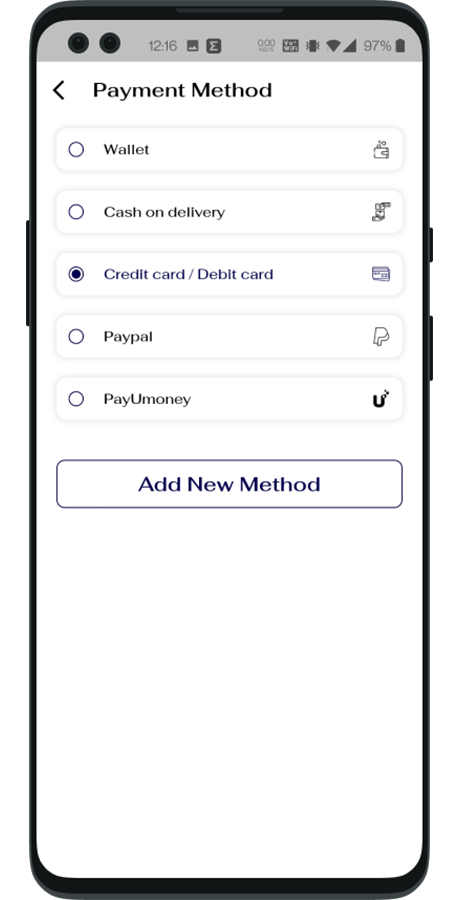This image depicts a digitally rendered graphic of a mobile phone characterized by a black outline and side buttons. The top of the phone features two camera lenses. The screen showcases a user interface with status icons for time, network connections, and battery life.

The displayed screen has a white background and is titled "Payment Method," accompanied by a backward arrow for navigation. Below the title, there are five 3D-styled boxes each representing different payment options: Wallet, Cash on Delivery, Credit/Debit Card, PayPal, and PayU Money. Each option is paired with an icon positioned to its right and radio buttons for selection.

The current selection, indicated in blue, is the Credit/Debit Card option. At the bottom of the screen, there's a button labeled "Add New Payment Method." While the layout is designed to mimic a real-life phone interface, the overall aesthetic does not achieve a realistic appearance.